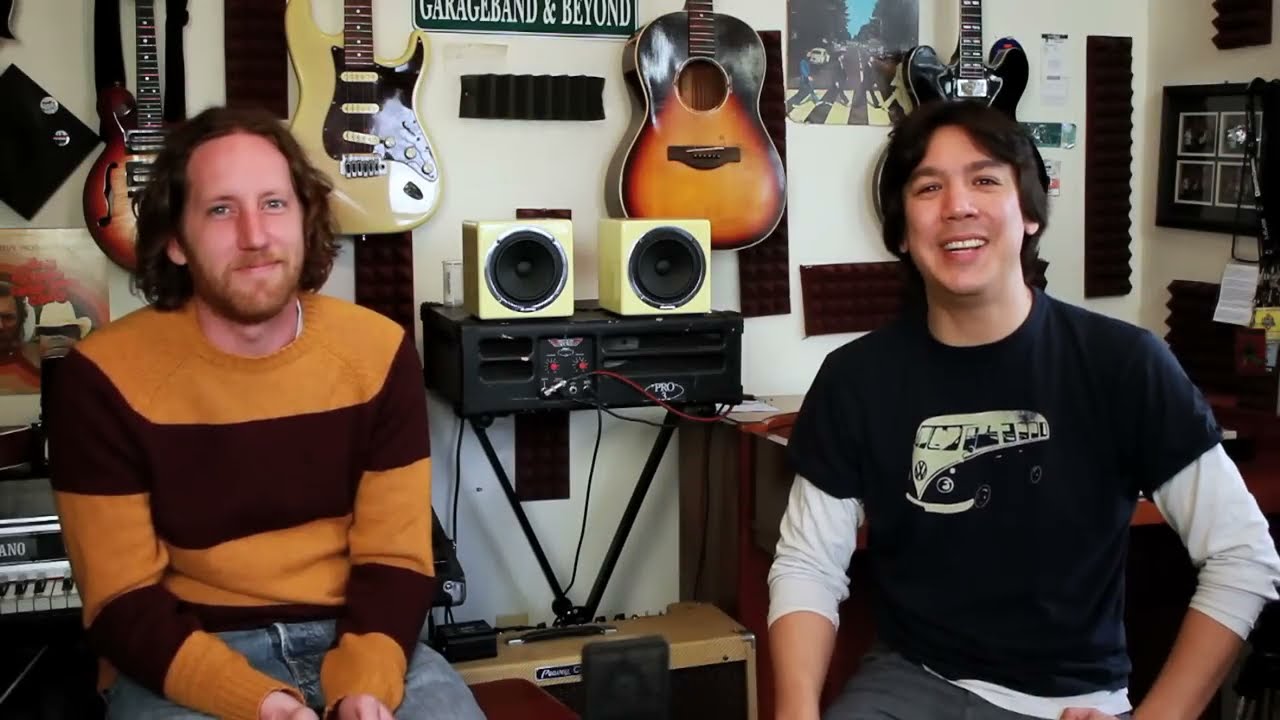In the photograph, two musicians are seated in what appears to be a recording studio, evidenced by a backdrop filled with various guitars, amplifiers, and soundproofing foam. The man on the left has fair skin with long, brownish-red hair and a light beard. He dons a distinctive sweater with alternating stripes of light mocha brown and rich dark chocolate, paired with blue jeans. He sits on a stool, facing forward with a subtle smile. To his right is a man with an olive complexion and slightly less long black hair. He is wearing a black t-shirt featuring an icon of a Volkswagen hippie van, over a white long-sleeve shirt, and gray jeans. Both men are smiling, with the man on the right showing a broader, jolly grin. The setting resembles a music-themed environment, with a visible sign reading "GarageBand and Beyond" and an album cover of the Beatles' "Abbey Road" contributing to the room’s artistic ambiance.